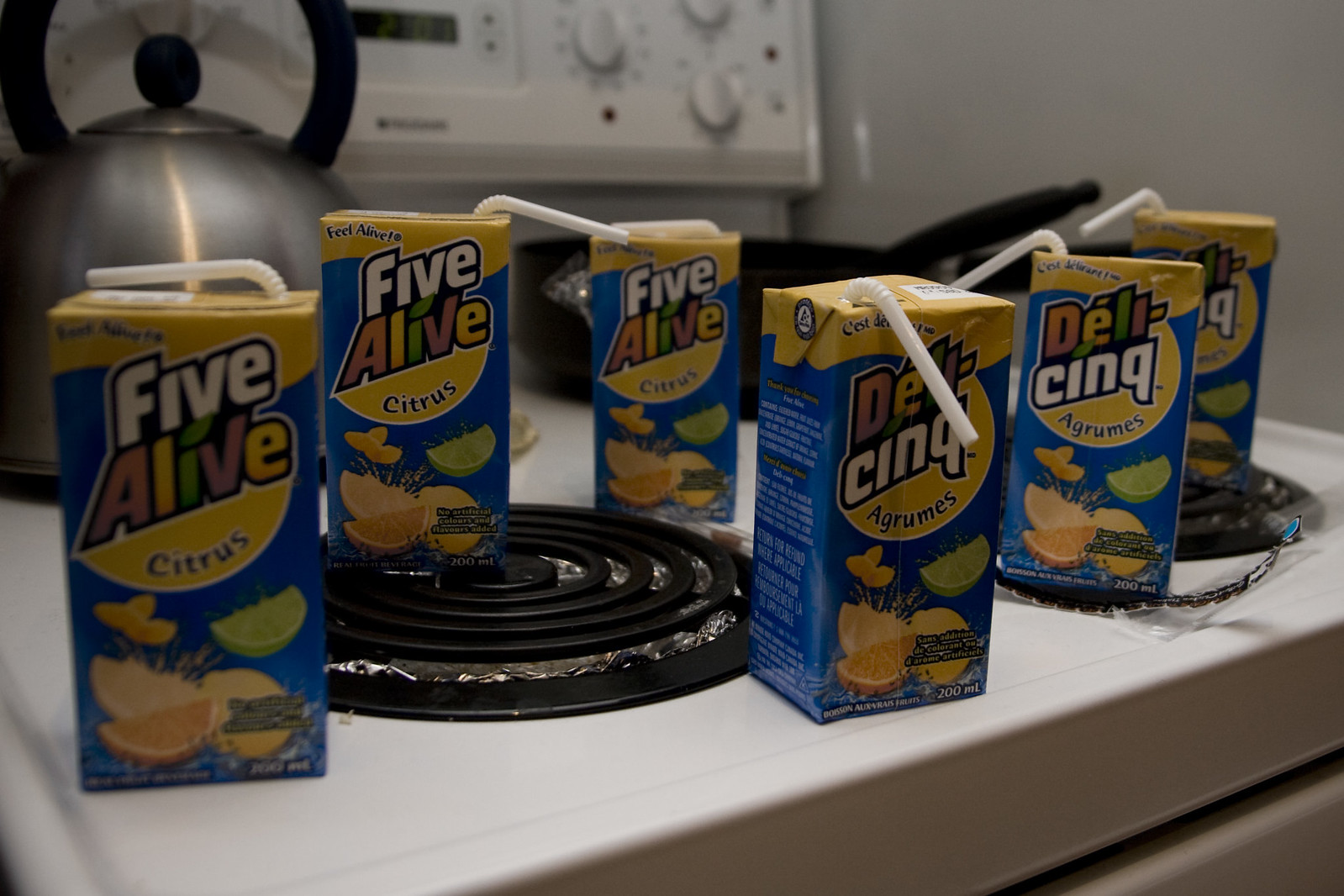This is a detailed photograph of five juice boxes arranged on a white stove, which features a silver tea kettle with a black handle and a black frying pan placed in the background. The image is taken slightly from the left-hand side, giving a partial view of the stove's black coiled electric burners and its interface, which includes various control knobs and a blurry information panel. 

The juice boxes are colorful, predominantly featuring blue backgrounds with yellow accents. They are branded "Five Alive" in all white letters for 'Five' and in multi-colored letters (red, yellow, green, red, and yellow) for 'Alive.' Three of these boxes also have a yellow block label stating "Citrus" and are adorned with images of oranges and limes. The remaining boxes showcase similar designs but in French, labeled "Déli Cinq Agrumes." All the juice boxes have white, bendable straws already inserted into the punch holes at the top, with the straws bent down slightly below the top edge of the boxes. 

Through a closer look, two of the juice boxes rest directly on the coiled burners, and the arrangement highlights a juxtaposition of vibrant juice packaging against the appliance's more subdued color tones and functional elements.